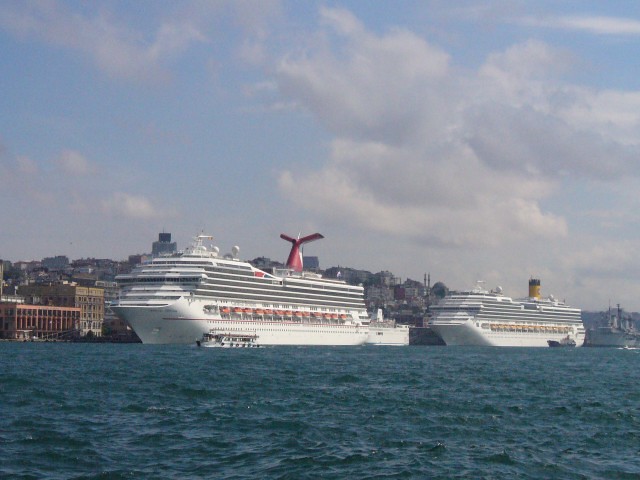This color photograph showcases a serene maritime scene featuring two large white ocean liners docked close to the shore. The calm aquamarine water in the foreground reflects the stability of the stationary vessels, while the deep bluish-gray hue of the ocean beneath them contrasts subtly. The docked cruise liners, adorned with red detailing and multi-layered decks, display distinct features: the one in the background has a smokestack, whereas the one in the front has a structure resembling a red wind turbine with two wings. Surrounding the grand liners are smaller craft, including a glass-bottom pleasure boat and a small powerboat, potentially a tugboat. The port is adjacent to a hilly cityscape with indistinct yet visible buildings. Above, a pale blue sky is dotted with cotton-like white and gray clouds, drifting low and spaced out over the horizon.